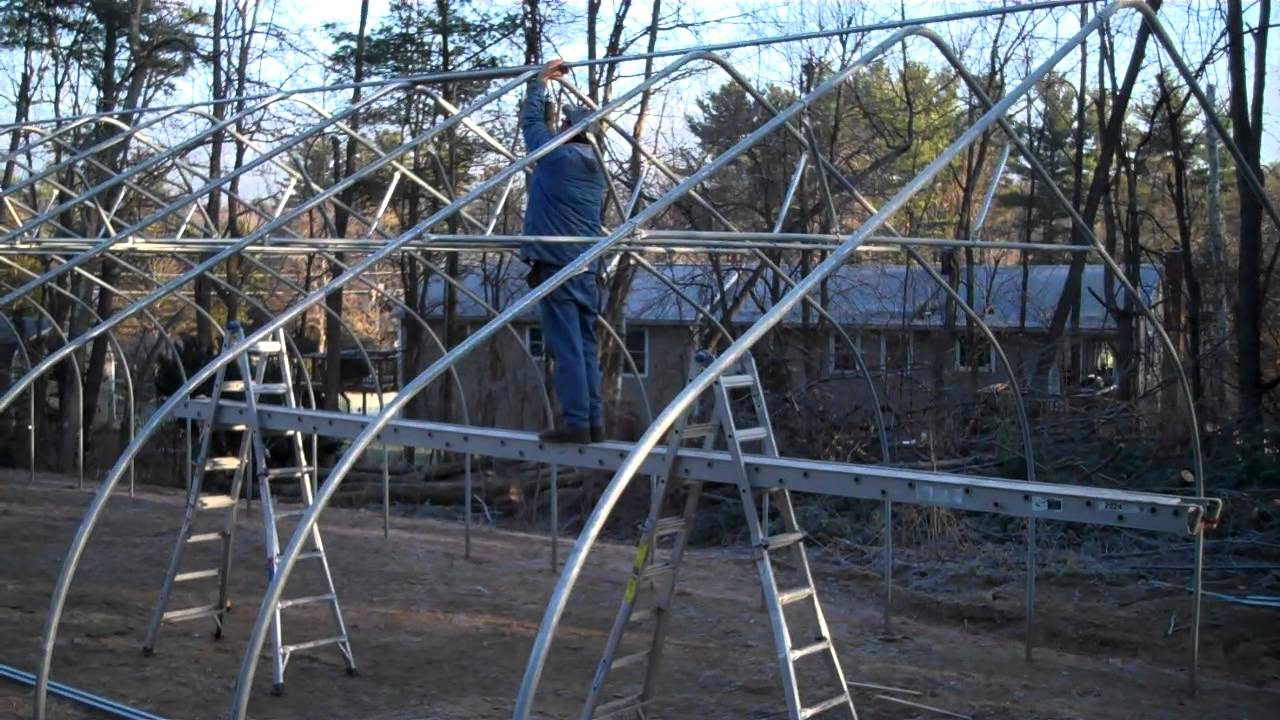The photograph depicts a man in the midst of constructing a greenhouse. The structure is clearly identifiable as a greenhouse by its A-frame, arched metallic sections which point at the top and extend diagonally down to the ground. Two ladders of the same height are positioned with a beam running horizontally between them, and the man stands securely on this beam. The man is dressed in blue work pants, a matching blue jacket, brown shoes, and a cap. His right hand is raised to the very top of the structure, appearing to tighten or fasten something, while his left hand steadies his position. The scene takes place in a wooded area, evident from the various trees surrounding the site. In the background, there is a small house, possibly a ranch or a mobile home, with a light gray roof. The sky is light blue, though the area where the man is working is shaded.